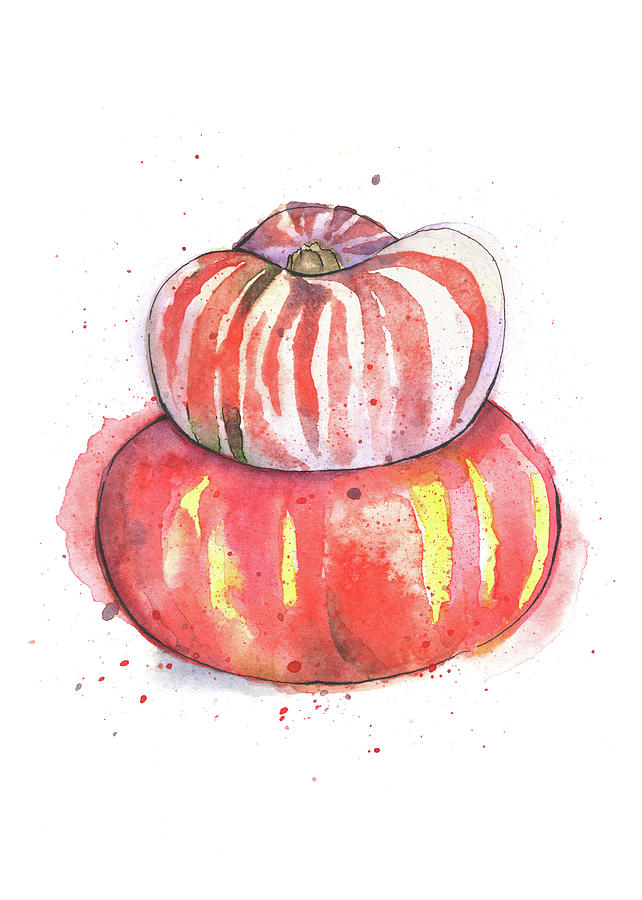In this image, two gourds or pumpkins are stacked on a white background adorned with tiny splashes of watercolor paint in various shades of brown and dark orange. The larger, bottom gourd is an orange-red color with distinctive yellow streaks indicating its segmented structure. It also features splashes and speckles of brown and red paint, some of which extend beyond its edges, creating an aura-like effect that appears to bleed out towards the top left and bottom right. Perched atop the larger gourd is a smaller, white gourd with vertical red streaks running down its sides and a visible brown stem on top. The painting, done in an expressive and slightly sloppy watercolor technique, brings a vibrant and lively feel to the piece, emphasizing its imperfections and artistic charm.